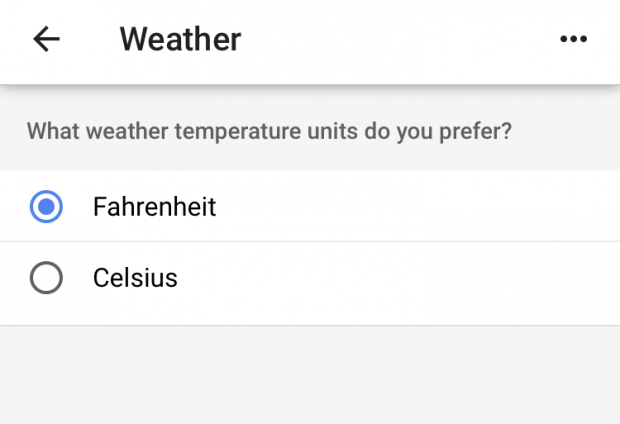The image shows a screenshot of the weather settings page on a smartphone. At the top of this page, there's a white rectangular bar extending from left to right, featuring a black arrow pointing left on the far left. Adjacent to the arrow, the word "Weather" is displayed with a capital 'W' followed by lowercase 'e-a-t-h-e-r'. On the far-right side of the top bar, there are three horizontally aligned dots.

Moving downwards, there's another gray rectangle containing the text "What weather temperature units do you prefer?" Below this prompt, there is a selectable option within a white rectangle. This option has a blue circle in the middle, indicating it is selected. The text "Fahrenheit" is positioned next to this circle and is fully spelled out in lowercase letters.

Further down, separated by a faint gray line, there is another option with an unselected white circle outlined in gray. The text "Celsius" appears next to this circle. Below this, another faint gray line separates the bottom section of the page, which is shown as a light gray rectangle.